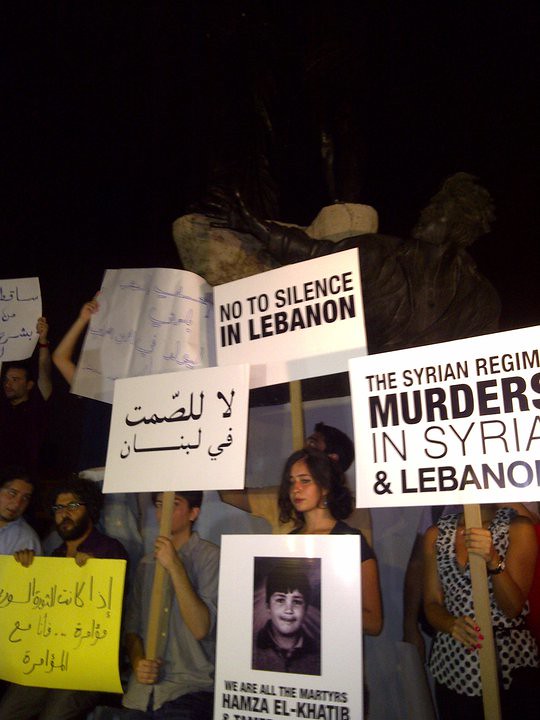This image depicts a nighttime protest rally likely held in Lebanon against the Syrian regime. In the lower third of the image, seven to eight people can be seen standing side by side, holding various protest signs with black text on white or yellow backgrounds. One prominent sign reads, "No to silence in Lebanon," held by an individual whose black hair is visible above the sign. Another sign states, "The Syrian regime murders in Syria and Lebanon," held by a woman wearing a black and white checkered blouse. Central in the image is a poignant sign featuring a photo of a young boy, Hamza al-Qatir, with the text "We are all the martyrs" beneath his picture. Several other signs display Arabic text. The protesters are dressed in light blue, black, and tan shirts. In the background, a light blue wall is partially visible, and the upper part of the image fades into darkness, indicating it is taken at night. To the left, there is a bronze statue of a man with his hand raised, though it is too dark to discern specific details. The overall scene captures the solemn and defiant mood of the protest.